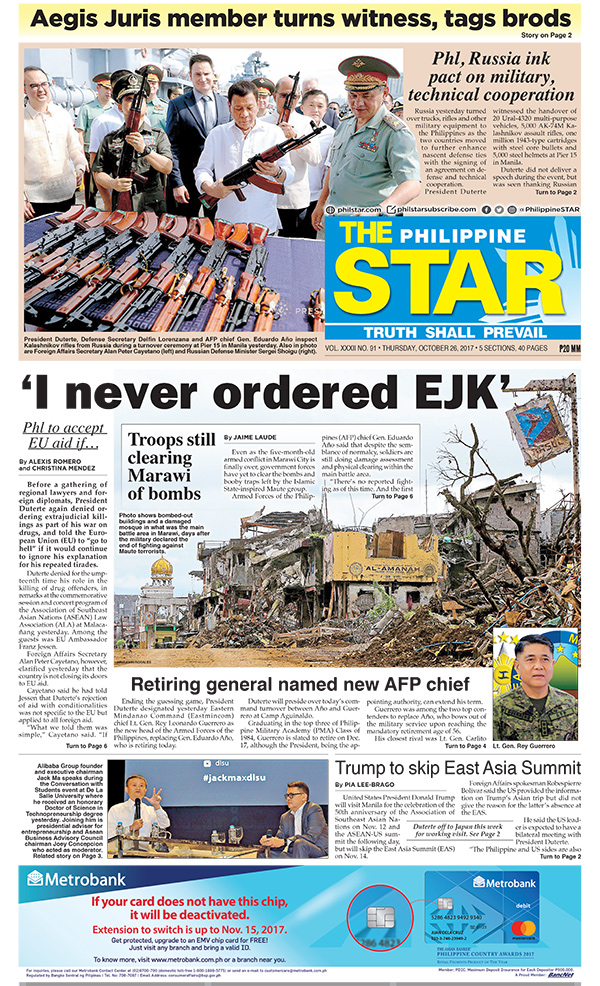This image depicts a newspaper page, likely sourced from a website, showcasing various articles and sections. At the top is a bold yellow headline reading: "Aegis Juris Member Turns Witness Tags Broads." Directly beneath this is a photograph showing several weapons laid out on a table, with a man in white holding one of the weapons, flanked by two men in uniform.

To the right of this photo starts an article titled "PHL Russia Inc. Pact on Military Technical Cooperation." Below this initial section is a blue banner featuring the publication's title, "The Philippines Star," accompanied by the motto "Truth Shall Prevail."

Under the banner, there's a white text box proclaiming "I never ordered EJK," leading into an article that runs down the left-hand column. At the center of the page is another article headlined "Troops Still Clearing Marawi of Bombs," accompanied by a photograph of blown-up houses and scattered debris.

Directly below this image is another headline, "Retiring General Named New AFP Chief," paired with a photograph of a young man in uniform. Adjacent to this, on the right, is an article titled "Trump to skip East Asia Summit," illustrated by a photograph of two people engaged in a debate.

The bottom section of the page is dominated by an advertisement for Metro Bank, featuring the bank's name in the top left corner and a dummy credit card on the right side. Finally, at the very bottom of the page, there's some copyright information.